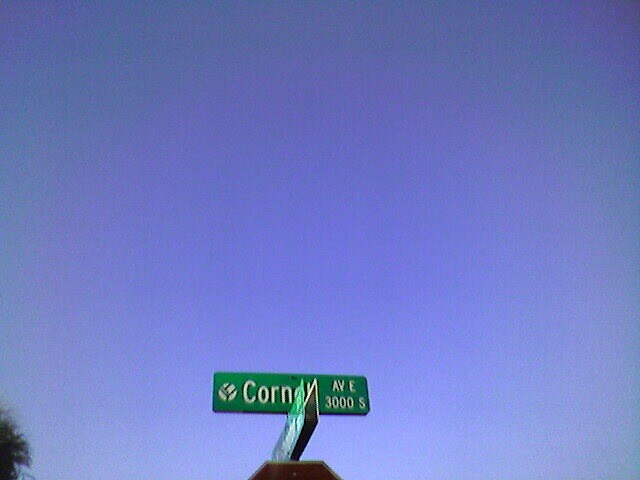This photograph, though blurry and pixelated, captures an urban scene on a sunny day. The image, taken from a low angle, partially shows a stop sign topped by additional street signs. The recognizable hexagonal shape of the stop sign is visible, with two green street signs mounted above it. The uppermost sign is legible and reads "Corn," likely part of "Cornell Avenue East 3000 S," and features a small logo next to the text. The second green sign is facing away, obscuring any readable information. Dominating the background is a vivid, clear blue sky, punctuated by the top of a tree branch in the lower left corner of the frame.